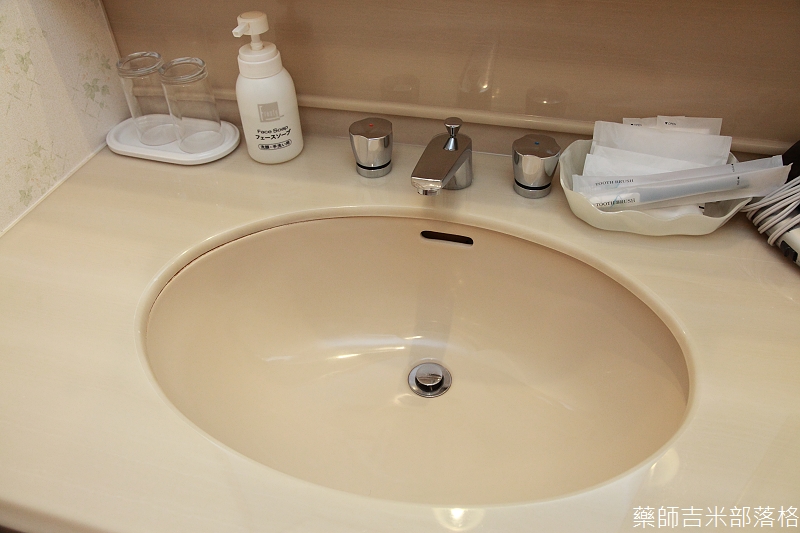This close-up photograph highlights a pristine bathroom sink area, seemingly part of a public restroom within a hotel, evidenced by the array of neatly arranged amenities. At the center is a cream-colored sink integrated into a matching countertop, exhibiting a harmonious, monochromatic aesthetic. The sink features separate hot and cold handles, along with a faucet equipped with a stopper. Adjacent to the sink on the right is a well-organized small stack, possibly consisting of folded napkins or informational pamphlets. Also partially visible to the far right is what appears to be a hair dryer or blower, partially cropped out from the frame. On the left side, a holder containing two transparent cups and an elegantly designed bottle of hand soap adds to the functionality and decor of the space. The sink area is immaculately clean and dry, bathed in bright lighting that enhances its spotless condition. Notably, the lower right corner of the image features Mandarin characters, suggesting location details or brand trademarks, further implying an international or Asian setting for this meticulously maintained facility.